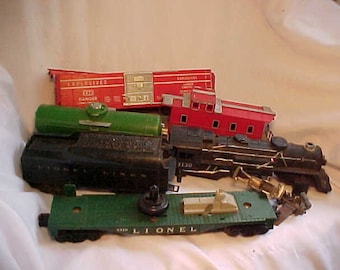This detailed, full-color indoor photograph, taken in natural light, features a staged display of a disassembled vintage Lionel toy train set. With a square orientation, the image shows the train parts neatly arranged atop a white cloth background. The centerpiece includes a classic black engine with gold detailing and a red caboose positioned slightly to the right with several windows visible. A black car, another red car, and a green tanker with a green lid are also part of the set, along with a green flatbed displaying the iconic "L-I-O-N-E-L" in white text. Notably, a red box with a beige center and illegible white text is placed at the top left corner, suggesting it may have originally housed some of these parts. The image encapsulates a nostalgic collection, reminiscent of childhood memories with realistic and representational product photography.